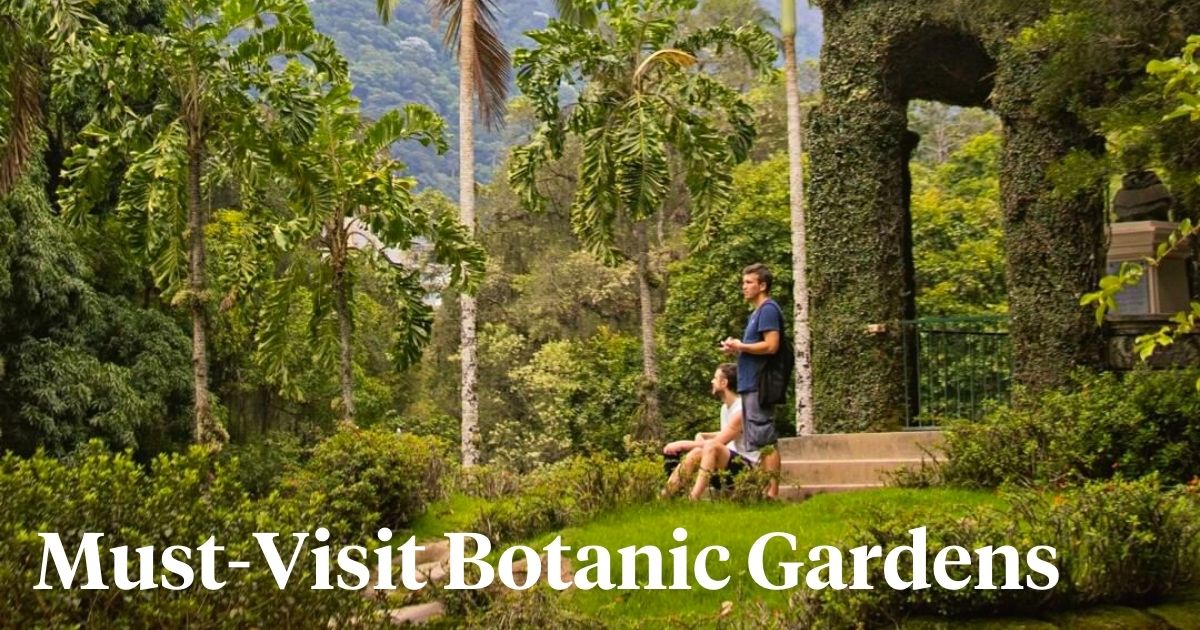This advertisement photo for the Botanic Gardens showcases a lush, verdant paradise filled with diverse vegetation. Dominated by tall, palm-like trees and dense greenery, the image is set against a mountainous background, suggesting a rich, natural setting. In the center-right of the image, a man dressed in blue shorts and a blue short-sleeved shirt stands gazing towards the left, while a woman in a white shirt and black shorts sits on stone steps, looking towards the mountains. The steps lead up to a vine-covered archway, hinting at a hidden pathway or entrance, and through the archway, a metal railing hints at an elevated platform or building. The lower portion of the image is carpeted in grass and bordered by bushes, amplifying the garden's lushness. Across the bottom, white text proclaims, "Must Visit Botanical Gardens," emphasizing the allure of this tranquil and inviting destination.